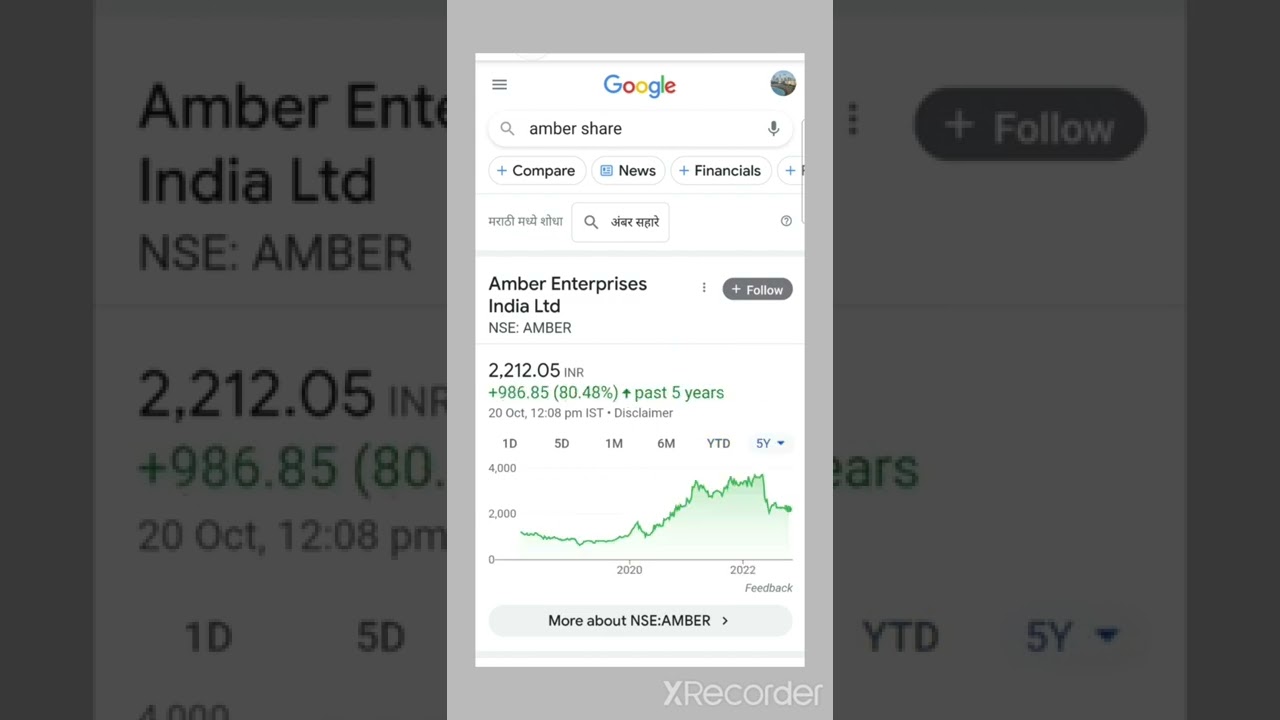This image is a composite of various elements revolving around the stock information for Amber Enterprises, India LTD, presented in a visually layered format. The primary background features an enlarged view of the stock details, which is partially obscured by a transparent black filter that adds depth and contrast to the image.

At the forefront, centrally positioned, is a focused screenshot of a Google search page displaying detailed information about the Amber Enterprises stock. In this screenshot:

- The Google logo is prominently displayed at the top, slightly off-center to the right.
- A user's profile icon is visible, indicating they are logged into their Google account.
- Below the logo is the search bar containing the text "amber share" in lowercase letters.
- Directly beneath the search bar are tabs labeled “Compare,” “News,” and “Financials,” though the rest of the content is truncated.
- Further down, the page clearly states "Amber Enterprises, India LTD, NSE: Amber."
- To the right of this text is a gray, inactive "Follow" button.
- The stock price is shown with its latest price change, along with the date and a graphical representation of the stock's performance over time.
- At the very bottom of this embedded screenshot, the phrase "More about NSE Amber" is centered, suggesting additional information is available on the subject.

In the bottom right corner of this overlay, the X Recorder logo in white signifies that the screenshot was captured using the X Recorder application.

Overall, this detailed and multi-layered image effectively combines various sources of stock information for Amber Enterprises into a single, comprehensive visual presentation.